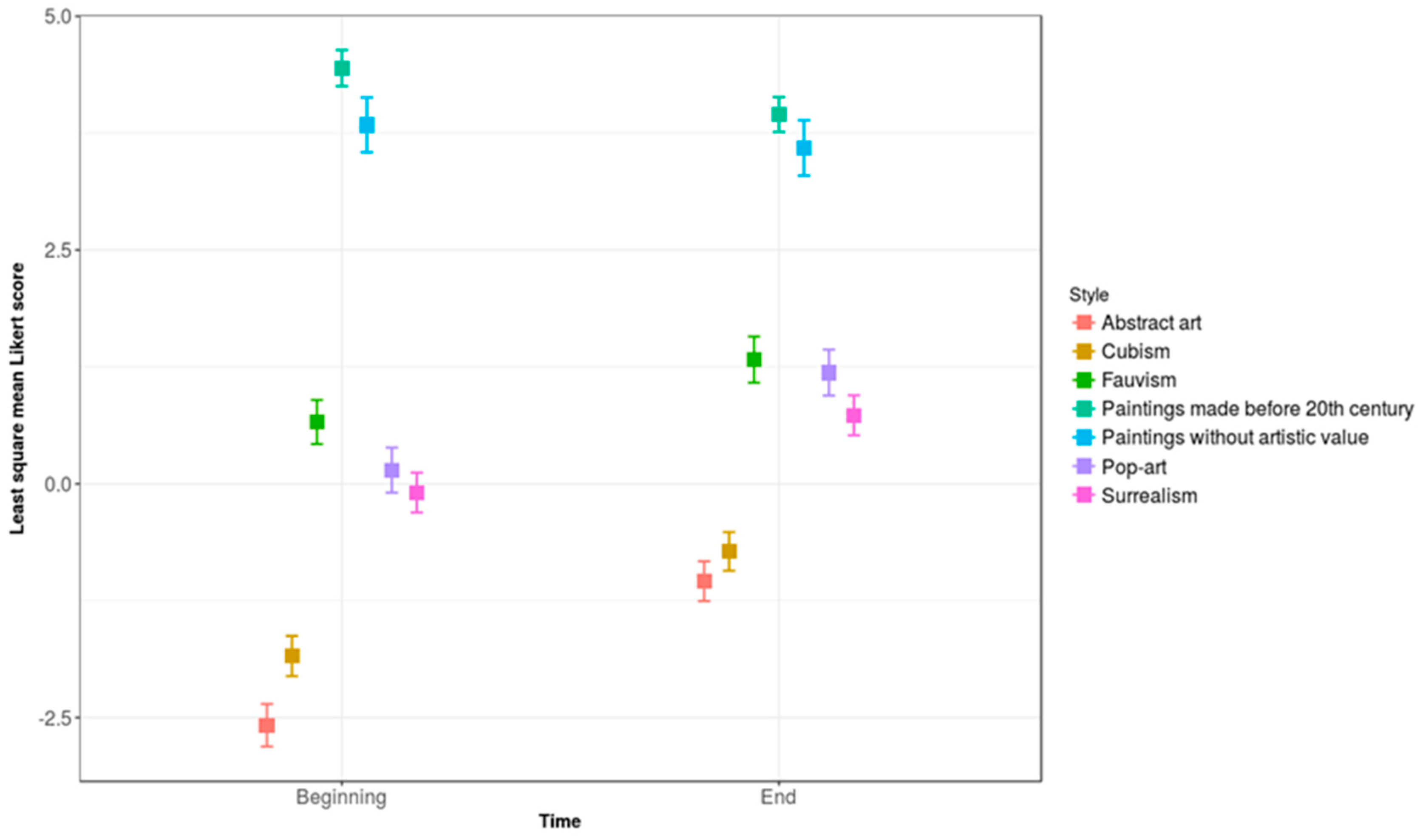The image displays a rectangular graph with a white background and a black outline, divided into a grid with three columns and seven rows. The horizontal axis at the bottom represents time, marked with "beginning" on the left and "end" on the right, both labeled in light grey. The vertical axis on the left indicates the least square mean Likert score, ranging from -2.5 to 5.0, with increments labeled at -2.5, 0.0, 2.5, and 5.0, vertically aligned from the bottom to the top.

To the right of the graph, there is a legend titled "style" that features a list of art styles denoted by specific colors. These styles include:
- Abstract art (orange)
- Cubism (yellow)
- Fauvism (green)
- Paintings made before the 20th century (teal blue)
- Paintings without artistic value (blue)
- Pop art (purple)
- Surrealism (pink)

The graph is populated with small colored rectangles corresponding to these styles, placed at various points to visually demonstrate their distribution over time.